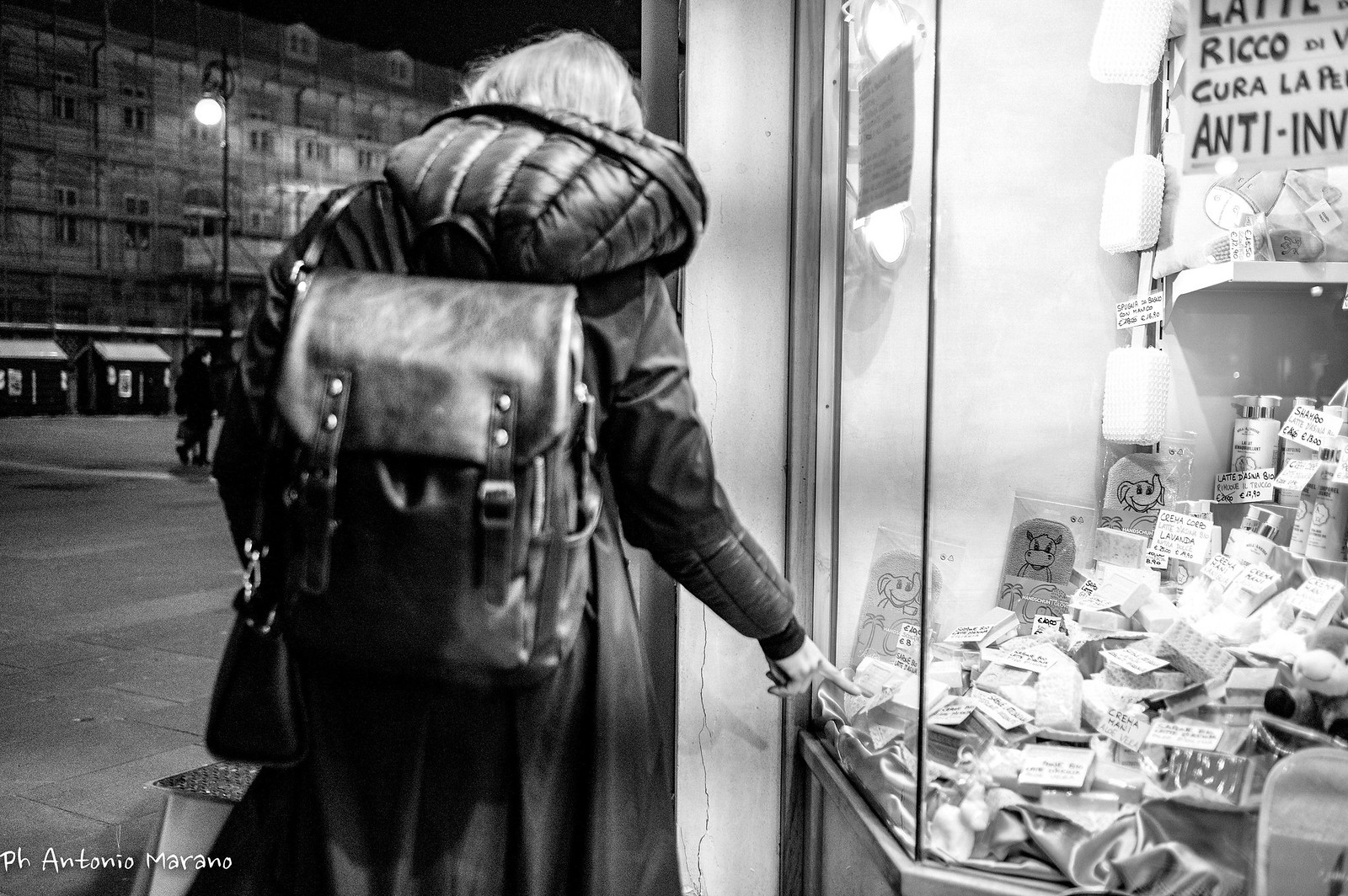This black-and-white nighttime photograph, titled "Photo Antonio Morano," captures a city scene where a woman, with lighter hair, is deeply engaged in window shopping. Wearing a heavy, long, black puffy coat with a hood, a black leather backpack adorned with two vertical straps and silver buckles, and a black purse with silver buttons on her left shoulder, she stands with her back to the camera. The woman's right arm is extended, her index finger gently touching the glass panel of a shop window to her right. The shop window displays a variety of items, including back scrubbers, cartoon elephants and giraffes, white tags, lotions, and an unreadable black sign. The sidewalk she stands on is adjacent to a large street, with a glowing streetlamp and small shed-sized buildings visible to the left. In the background, a distant wall of buildings is partially seen through the dim illumination, adding depth to the urban night scene. At the bottom left-hand corner, the photographer's name, Antonio Murano, is etched in white font, adding a personal touch to the atmospheric image.